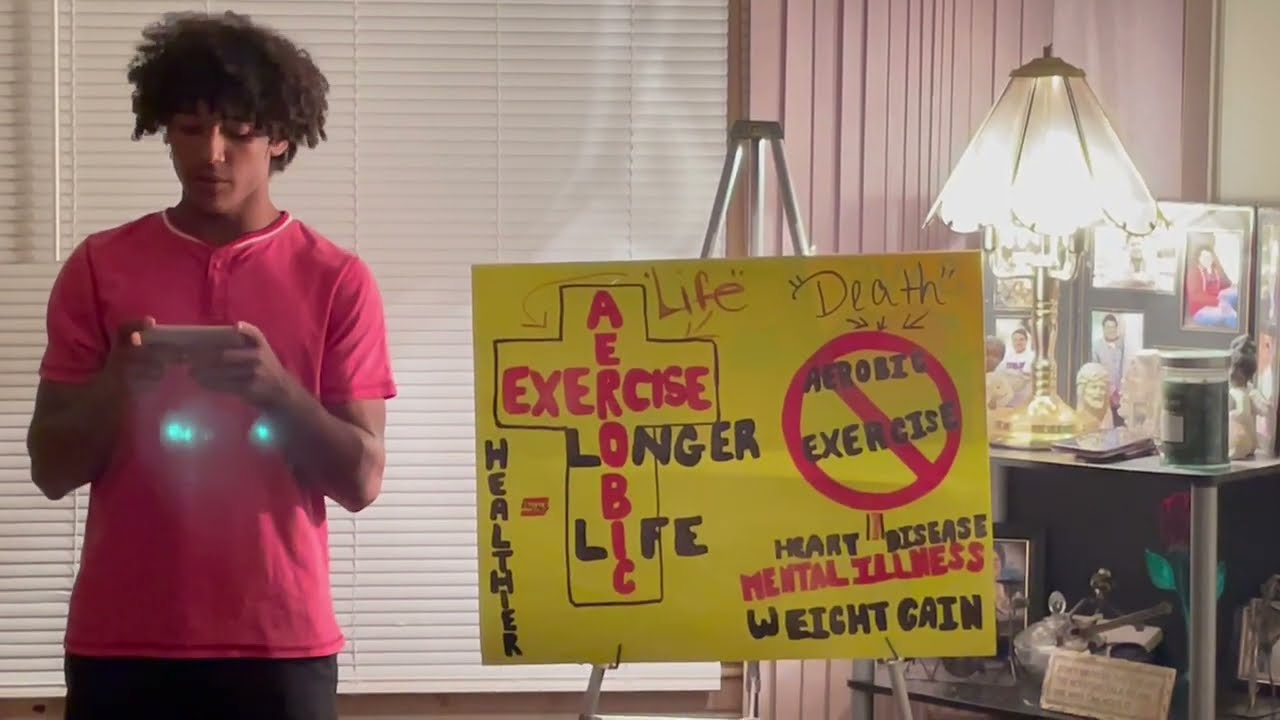In a cozy, warmly-lit room with white Venetian blinds covering a window and a brown wall adjacent to it, we see a young Hispanic or African-American teenager, possibly in high school or college, standing and engrossed in a smartphone he holds in his hands. He sports a vibrant pink, short-sleeved t-shirt with a button-down chest and black trousers. His hair is tightly coiled and poofy, adding to his relaxed yet focused demeanor. To his right, prominently displayed on a tripod easel, is a bright yellow, hand-drawn sign promoting the benefits of aerobic exercise. The sign features various texts in bold red and black, highlighting phrases such as "Aerobic Exercise," with a red cross through it, and "Longer Life," "Heart Disease," "Mental Illness," "Weight Gain," and "Death," indicating a life-death contrast associated with aerobic exercise. To the right of this sign, there's an antique table adorned with an old-fashioned lamp and several framed photos, adding a nostalgic touch to the setting. Blue lights from an unseen source cast a soft glow on the teenager’s t-shirt, enhancing the intimate ambiance of the scene. The overall setting suggests an earnest effort to advocate for a healthier lifestyle through aerobic exercise.